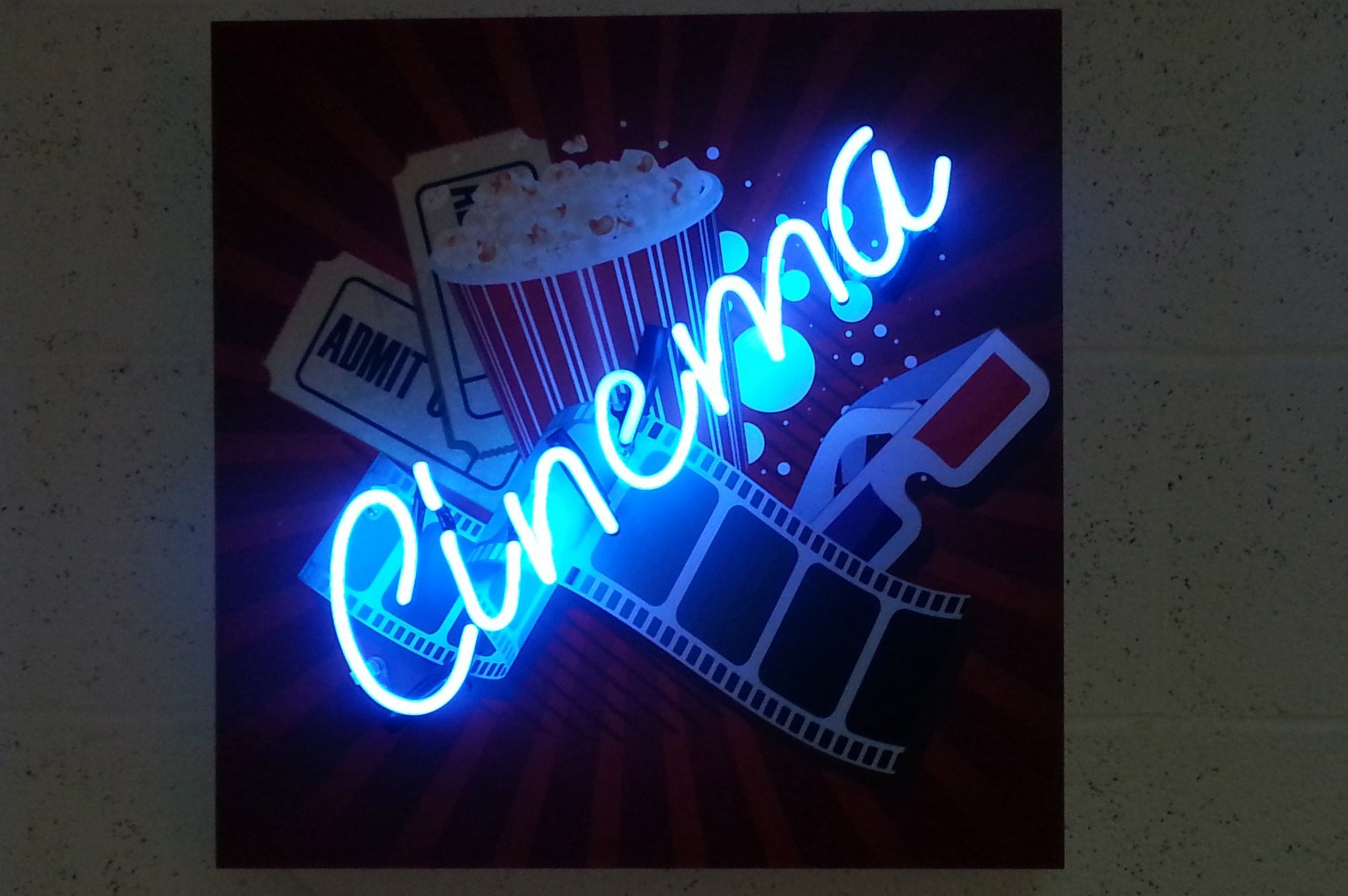In this photograph, set against a muted gray background, a striking neon sign spells out "CINEMA" in a diagonal, cursive-like font—white neon lighting that cuts through the scene from the bottom left to the top right. The sign is illuminated brightly, casting a glow over an array of classic cinema-related items beneath it. Behind the neon letters, a roll of movie tickets is visible, with one clearly marked "ADMIT." A red-and-white striped bucket of popcorn sits prominently, kernels spilling out, accompanied by a pair of retro 3D glasses with blue and red lenses. Interspersed amongst these items are aqua blue bubbles subtly glowing in the background. This collage captures the nostalgic essence of movie-going, enveloped in the cool, luminescent light of the neon sign. The entire set-up, with its vivid elements and darkened backdrop, creates a captivating, almost iconic movie theater logo.